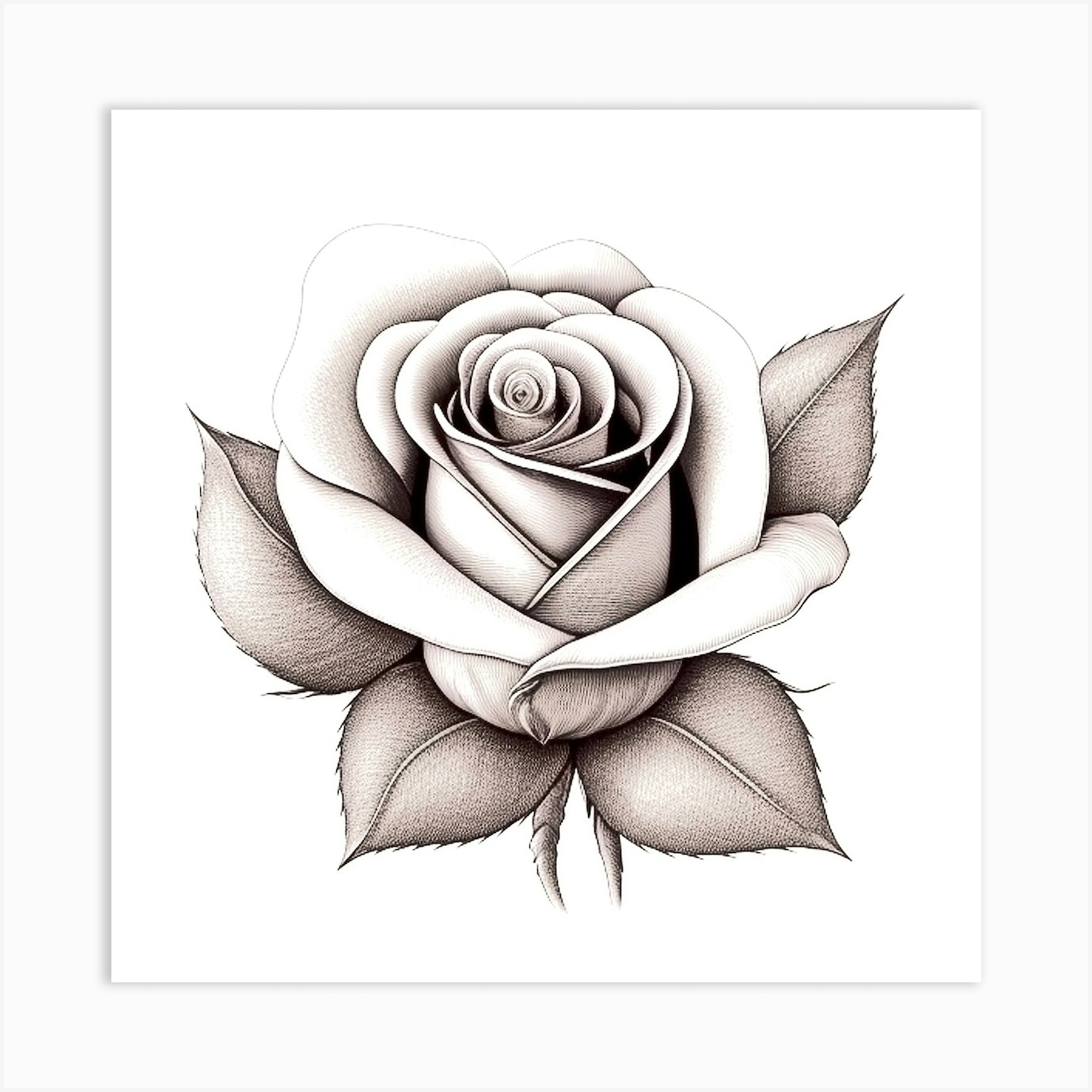This detailed illustration of a rose, executed in sepia tones with a pen-and-ink technique, boasts exquisitely fine strokes and intricate shading, enhancing its texture and depth. The centerpiece is a blossoming rose, not fully open but at the peak of its bloom, showcasing a concentric arrangement of petals with some gently folding back to reveal the layered core. The rose is framed by four serrated leaves, two on each side, and features an unusual split stem. The meticulous linework, shading, and shadows intricately define the petals and leaves, highlighting the contrast between the velvety inner petals and the darker, textured outer petals, as well as between the leaves and the petals. Set against a stark white background, the artwork itself casts a delicate drop shadow, creating a slight elevation effect, reminiscent of a posterized image. This illustration, resembling a potential tattoo design or clip art, utilizes a unique line texture technique where both fine lines and minuscule squares build the shades of gray and white, ensuring each detail stands out in high contrast.